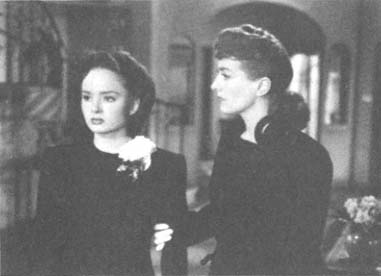This image is a screenshot from an old black-and-white movie, possibly from the 1940s or 1950s. It depicts two women standing together in the room of a Victorian-style house with high ceilings and archway doorways. Both women are wearing black long-sleeved dresses, suggesting they might have been to or are going to a funeral. The woman on the left, who has short black hair styled past her chin and combed back, is looking to the left-hand side with a scared and concerned expression. She also has a white flower or corsage on her shoulder. The woman on the right, with her hair tied back in a ball behind her neck, is gazing at her companion with a concerned look and has her arm around the left woman's arm, providing comfort. The overall atmosphere is somber, reflective of the era and style of classic films reminiscent of Bette Davis's time.